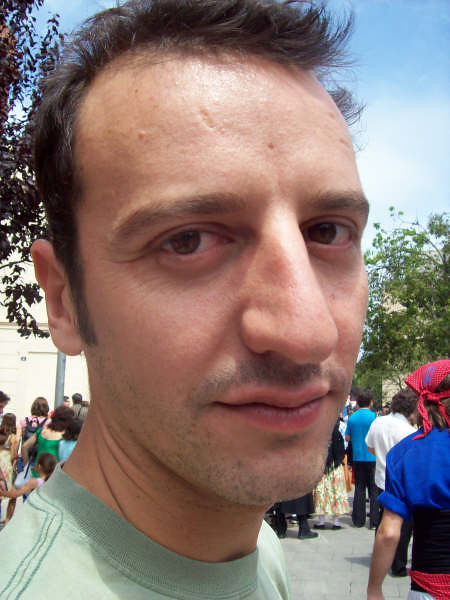In this selfie, a man, likely in his early 30s, is outdoors with a slight smile on his face. He has short, thinning brown hair that’s about an inch long on top and a quarter of an inch on the sides, with visible sideburns and facial stubble. He wears a light green t-shirt. Behind him, a large group of people can be seen, some wearing t-shirts and others in long dresses or gowns, standing on what appears to be a tile or cement ground. The sky above is a clear, vibrant blue with minimal cloud cover, and there's a green tree visible to the right. One notable person in the background wears a distinctive red do-rag, a blue shirt, and red pants, making them stand out in the crowd. The overall setting suggests a possible festival or outdoor event.